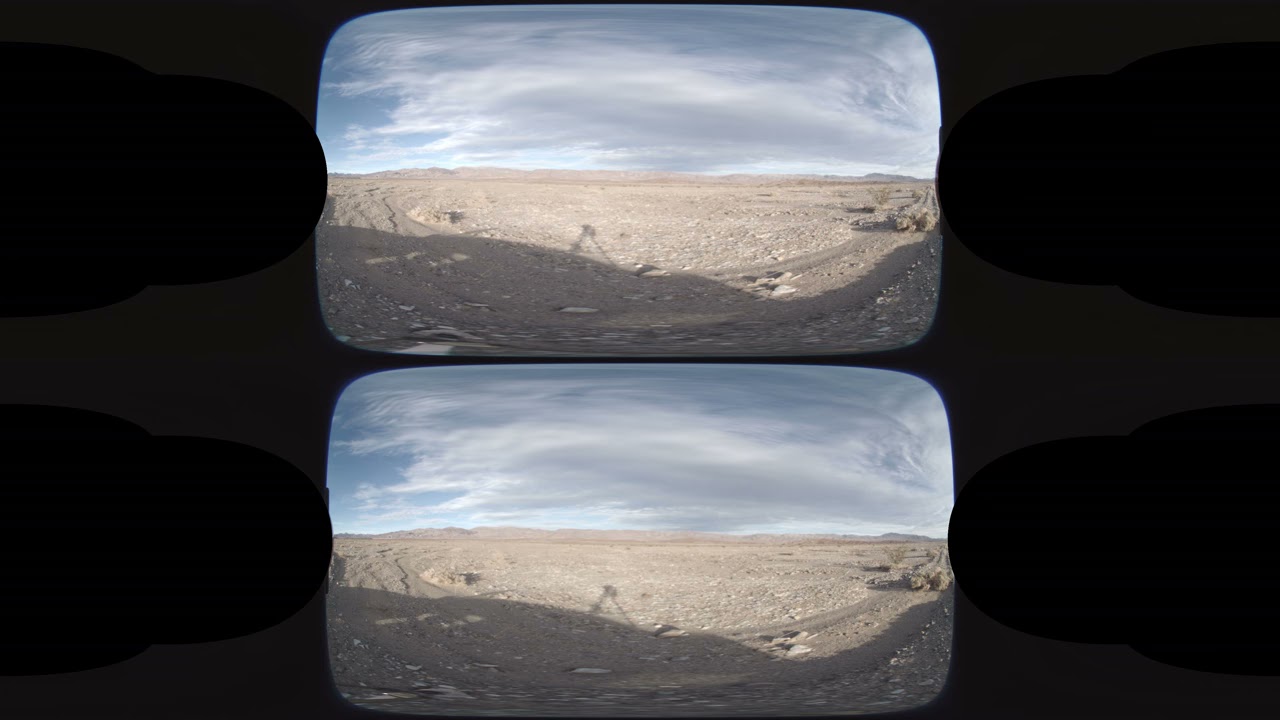A black rectangular frame contains two identical images stacked vertically, each capturing a vast, barren landscape. The expansive, empty area is covered in beige and brown sand interspersed with rocks and stones. Shadows are cast upon the soil, hinting at the intensity of the sun’s rays in this daytime scene. The open terrain extends to the horizon, where a pile of boulders is visible in the distance on the right side. Beyond this, a series of hills and mountains form a faint, far-off backdrop. Above the horizon, the sky is a clear blue, adorned with swirling gray and white clouds.